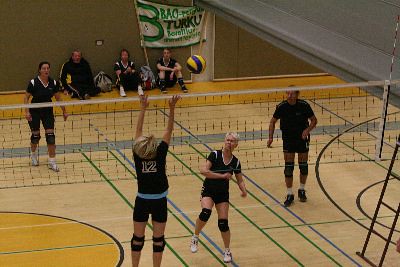The image captures a high-energy women's volleyball game with a mixed presence, featuring both men and women players on the court. The scene is set indoors, with a dark brown wall serving as the backdrop. On the near side of the net, two blonde women, each clad in black volleyball attire, are actively engaged. One has just hit the yellow and blue striped ball upwards, and her partner, donning a jersey with the number 12, appears ready to make the next move. Both players sport black knee pads. A lone man, also equipped for play with knee pads and black sneakers, shares this side of the court, his role as either a player or coach unclear. Across the net, a solitary woman stands poised in white sneakers, ready to respond. In the background, three spectators are seated against the wall, intently watching the match. Between them, a banner displaying white and green text in a foreign language adds a touch of ambiance to the setting.